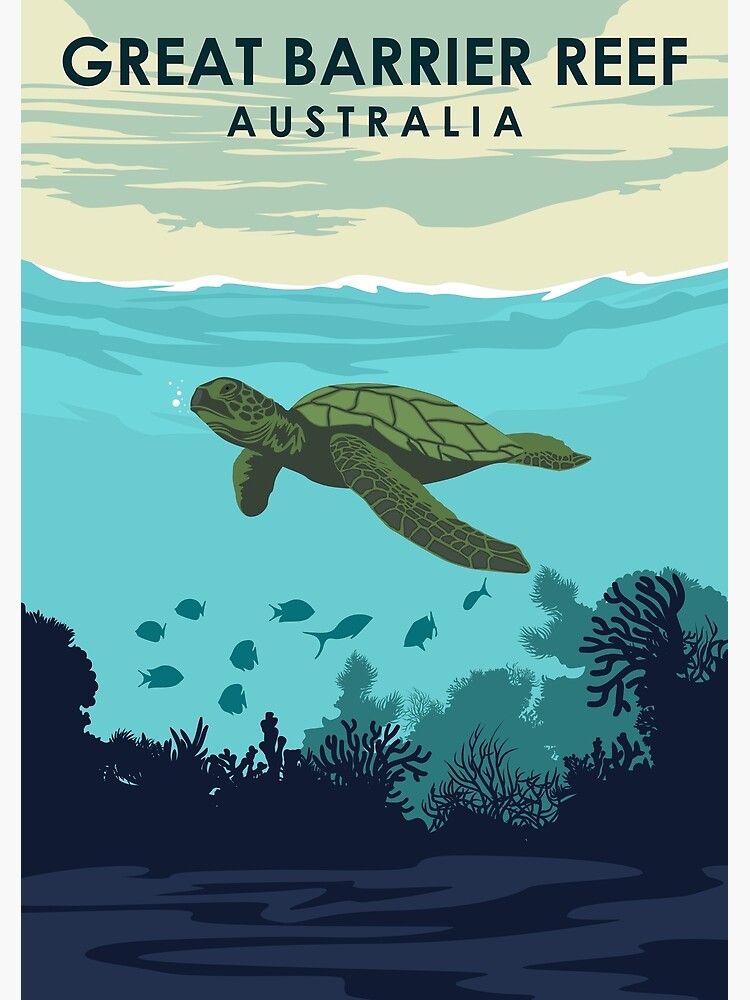This poster promotes the Great Barrier Reef in Australia, showcasing an artistic representation of the vibrant marine life. Central to the composition is a green sea turtle, depicted in shades of army green, floating gracefully near the surface of the turquoise water. The water itself transitions from the light blue waves at the top to deeper blue tones towards the ocean floor. Above the water, the sky is painted in light yellow hues with streaks of gray clouds. Text at the top reads "Great Barrier Reef Australia" in dark blue, almost black, adding to the promotional feel of the poster.

Beneath the turtle, the ocean teems with life, illustrated in minimalist style. Fish, resembling goldfish crackers in shape and colored in darker blue hues, swim among silhouettes of coral and sea plants that populate the sea floor. These elements are presented in varying shades of blue, creating a harmonious underwater scene. The drawing style of the poster is animated and minimalist, yet detailed enough to capture the essence of this iconic Australian ecosystem.